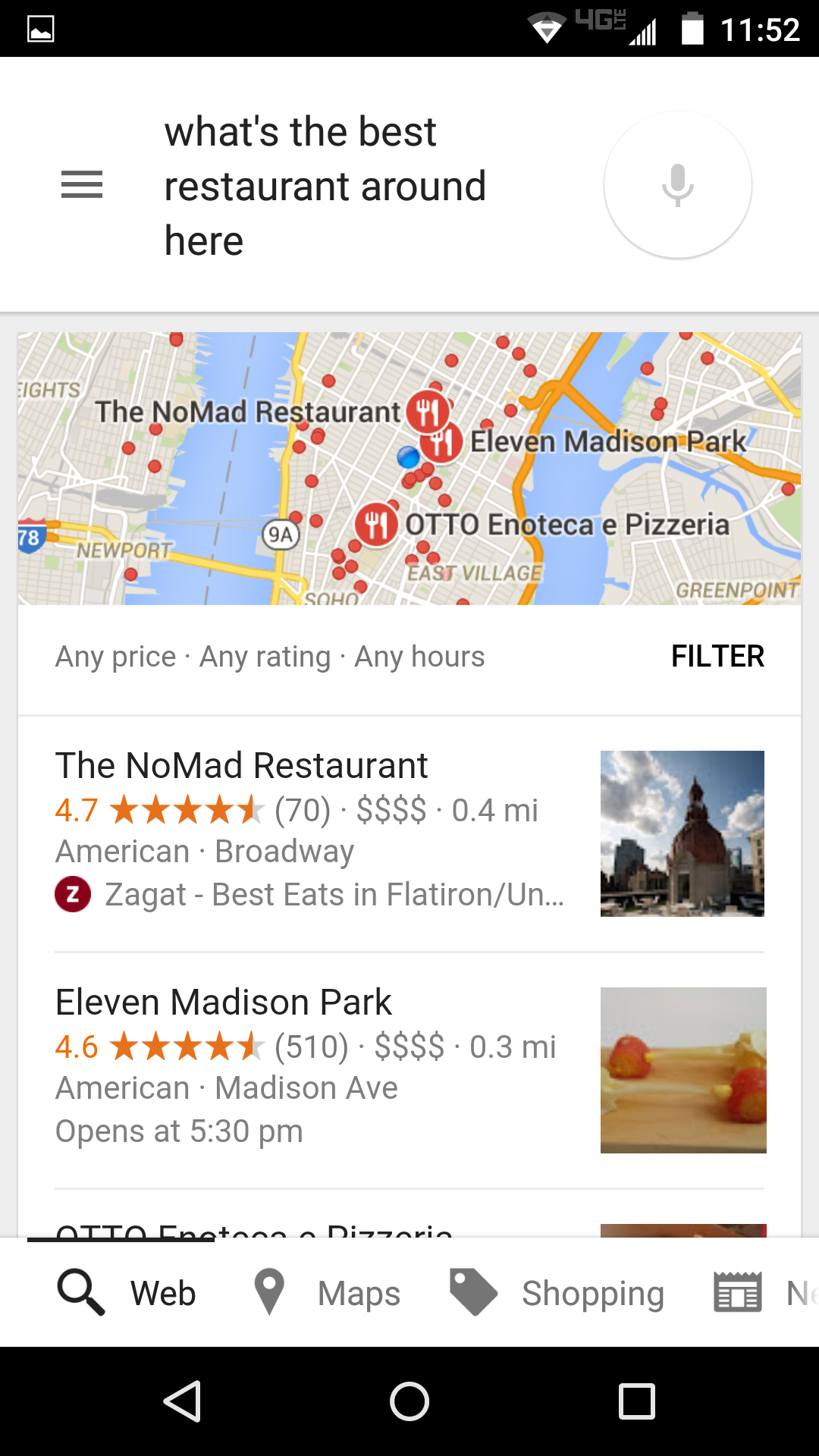In this image, a person is seen on their phone, evidenced by the screenshot icon at the top left corner. On the far right, icons display a 4G LTE signal, Wi-Fi strength, battery level, and the current time of 11:52. The phone's screen shows a white-background search page where the user has asked, "What's the best restaurant around here?" via voice input, indicated by the microphone icon next to the text.

Below the query is a map featuring locations such as Newport, Greenpoint, East Village, and Soho, suggesting the area is Manhattan. Highlighted on the map are three pinpointed restaurants: The Nomad Restaurant, Eleven Madison Park, and another place barely visible named OTTO Enoteca Pizzeria.

Further details about the restaurants are listed under the map. Filters at the top indicate options for any price, any rating, and any hours. The Nomad Restaurant and Eleven Madison Park both have four-dollar signs, denoting high expense. The Nomad Restaurant is categorized under "American Broadway" and noted as a Zagat Best Eat in the Flatiron district. Eleven Madison Park is specified as "American Madison Avenue," opening at 5:30 PM. Small thumbnail images of the locations accompany the text listings, providing a visual clue to their settings.